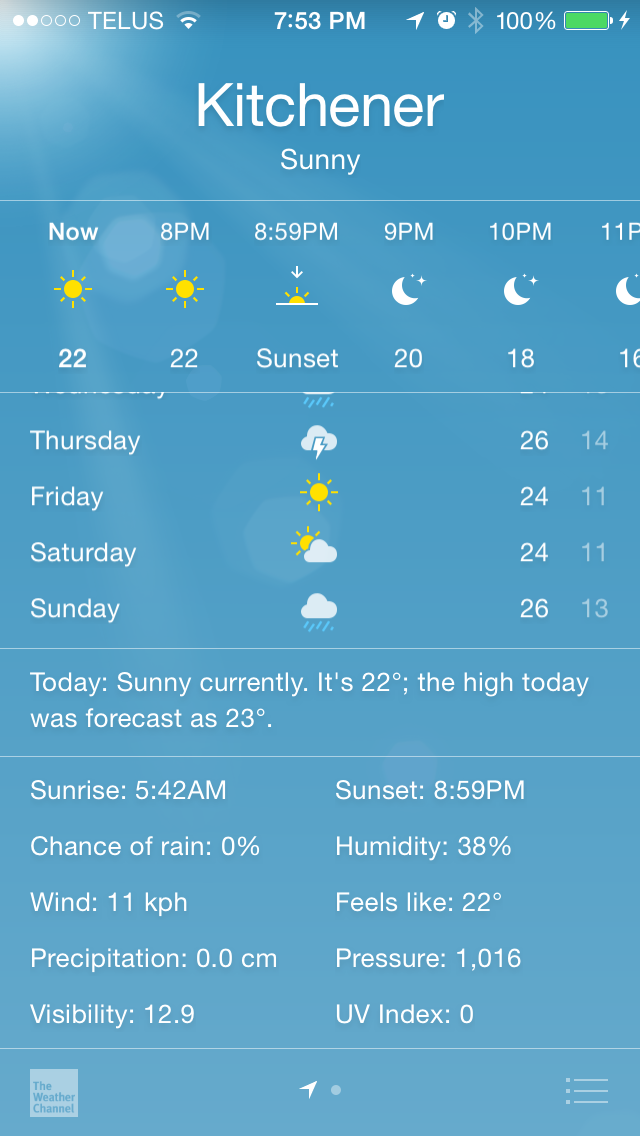In this detailed weather app screenshot, we see a modern smartphone interface against a blue background with white text. At the top-left corner, the time is displayed as 7:53 p.m. The phone signal shows 100% with the location set to Kitchener, which currently has sunny weather. Below this, there is a light blue line separating sections. 

In white text, the current weather condition "Now" is highlighted with a yellow sun icon, indicating a temperature of 22°C at 8 p.m. An arrow points downward, denoting that the sun is setting, which will occur at 9 p.m. Following the sunset, the forecast shows a moon and stars icon for 10 p.m. at 20°C, 11 p.m. at 18°C, and midnight at 16°C.

A subsequent line divides this information from the multi-day forecast, displaying:
- **Thursday:** Clouds with lightning at 26°C during the day and 14°C at night.
- **Friday:** Sunny with a high of 24°C and a low of 11°C.
- **Saturday:** Partly sunny with the sun peeking behind a cloud, with temperatures reaching up to 24°C during the day and 11°C at night.
- **Sunday:** Cloudy with temperatures of 26°C during the day and 13°C at night.

A small line beneath this section leads to today's detailed forecast, showing "Sunny" at 22°C currently. The high was forecast at 23°C. Additional weather specifics are also provided:
- **Sunrise:** 5:42 a.m.
- **Sunset:** 8:59 p.m.
- **Chance of Rain:** 0%
- **Humidity:** 38%
- **Wind:** 11 kph
- **Feels Like:** 22°C
- **Precipitation:** 0.0 cm
- **Pressure:** 1,016 mb
- **Visibility:** 12.9 km
- **UV Index:** 0

Another line separates these details from the weather source, credited to The Weather Channel, accompanied by a white arrow pointing up and to the right. A white dot, followed by three horizontal lines with circles in front of them, completes the interface.